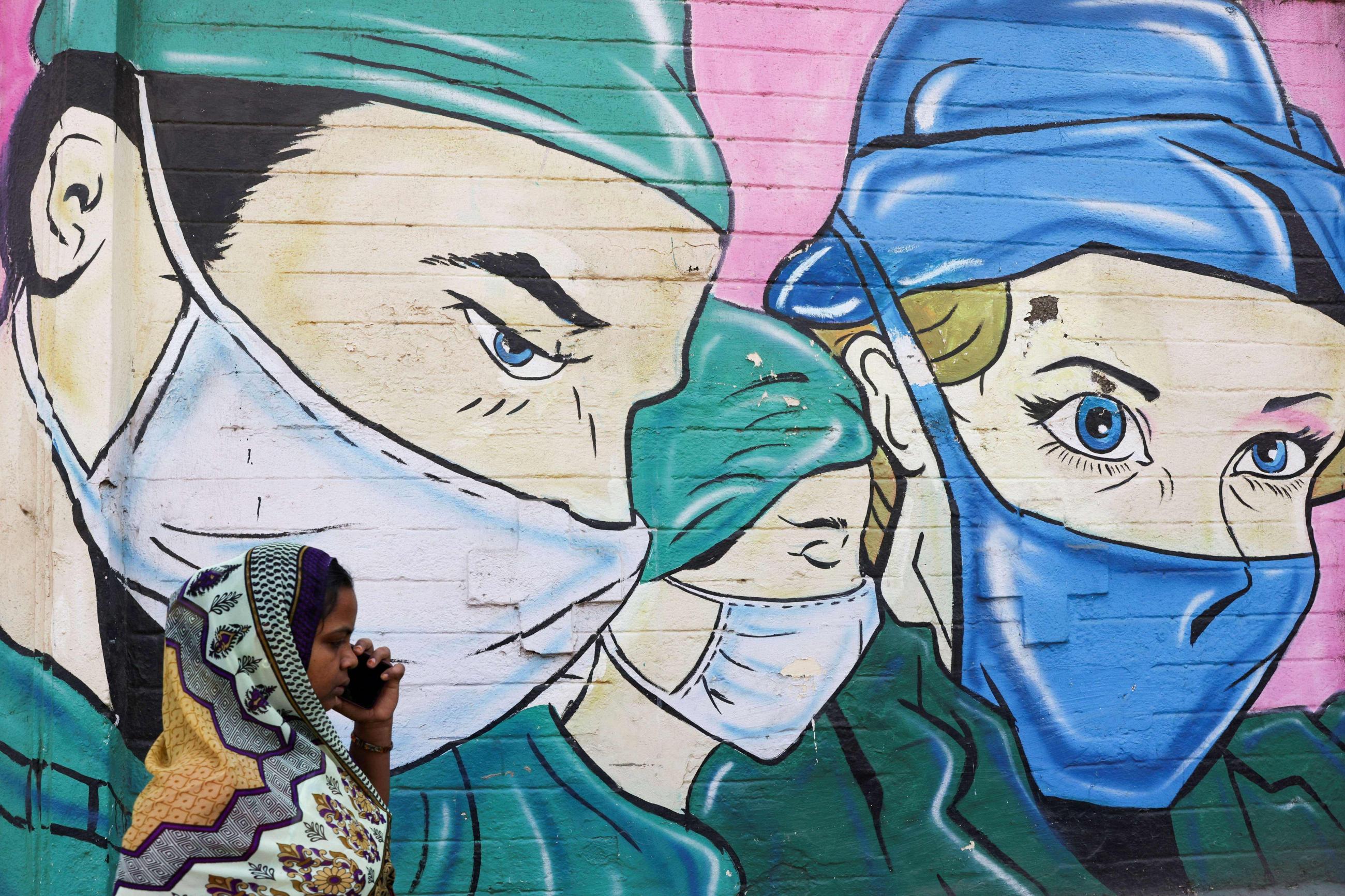The photograph captures a striking scene of a dark-skinned woman with black hair, walking to the right while talking on a smartphone held to her ear. She is adorned in a multicolored hijab that features a mix of white, blue, and orange hues, with various intricate designs and shapes. The background is dominated by a vibrant pink mural portraying close-up images of healthcare workers. On the far left, a Caucasian man with brown hair, blue eyes, and a green scrub cap and scrub top is seen. Next to him, a woman with her eyes closed, seemingly in deep thought, is depicted in similar green scrubs and head covering, with a light blue surgical mask. To her right stands another woman with gold-colored hair and striking blue eyes, distinguished by her blue scrub cap and matching blue mask. The overall mural embodies a sense of urgency and dedication among healthcare professionals, providing a vivid backdrop to the woman engrossed in her phone conversation.